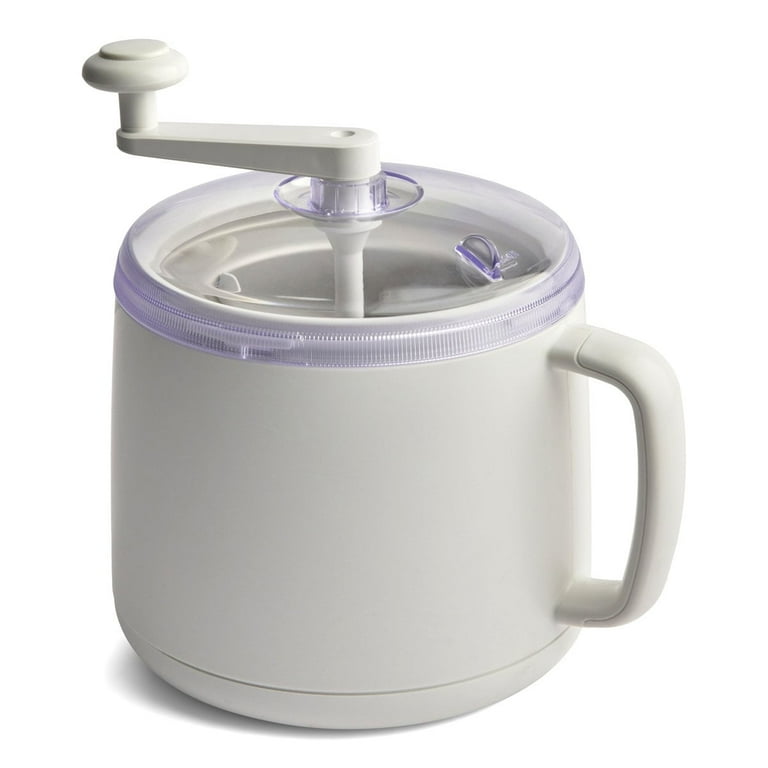The image features a white, ceramic-like container reminiscent of a coffee mug, equipped with a handle on the right. The top of the container is fitted with a clear plastic lid that has ridges around its edge. Emerging from the center of the lid is a white, cylindrical tube with an attached hand crank. This crank, constructed from a sturdy plastic, has a horizontal handle extending into a round disc shape, designed to be turned in a circular motion. The background of the image is a plain white, highlighting the main object with no distractions. The exact function of the device is ambiguous, but it could be used for grinding coffee beans or perhaps making ice cream or churning butter, given its crank mechanism and container design.